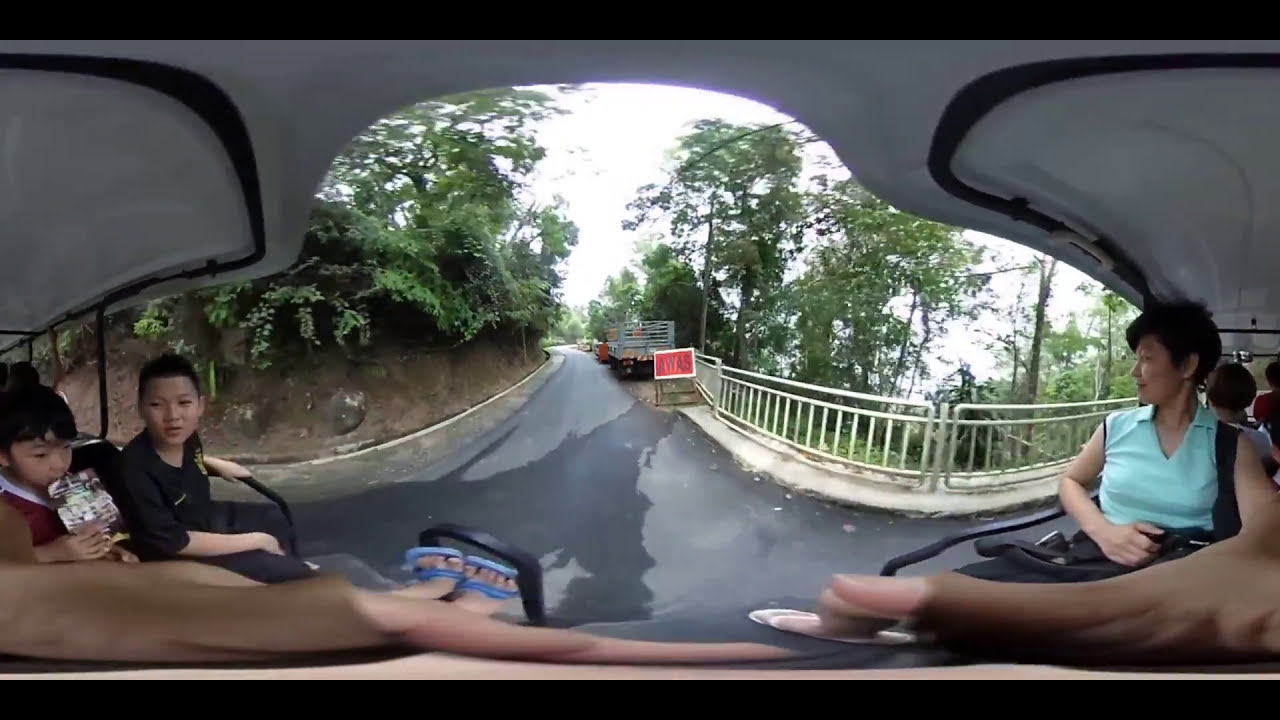The image depicts an amusement park ride, likely a tram or trolley with a white interior and black trim, capturing the view from a mounted camera inside the vehicle. Passengers, seated on either side facing each other, include a young girl in a red and white dress drinking from a silver pouch, a boy in a black t-shirt, and an older woman in a blue shirt with short hair and her arm resting on her lap. The scene outside shows a road ascending a steep hill flanked by steep dirt walls on one side with greenery, and a silver fence on the other side. There is also a red and black sign in the middle of the road and a truck with a trailer parked on the side. The clear daytime setting is brightly lit, highlighting scattered trees on small hills surrounding the fenced area. A person wearing blue sandals and possibly the hand of the person taking the picture are also visible in the frame.